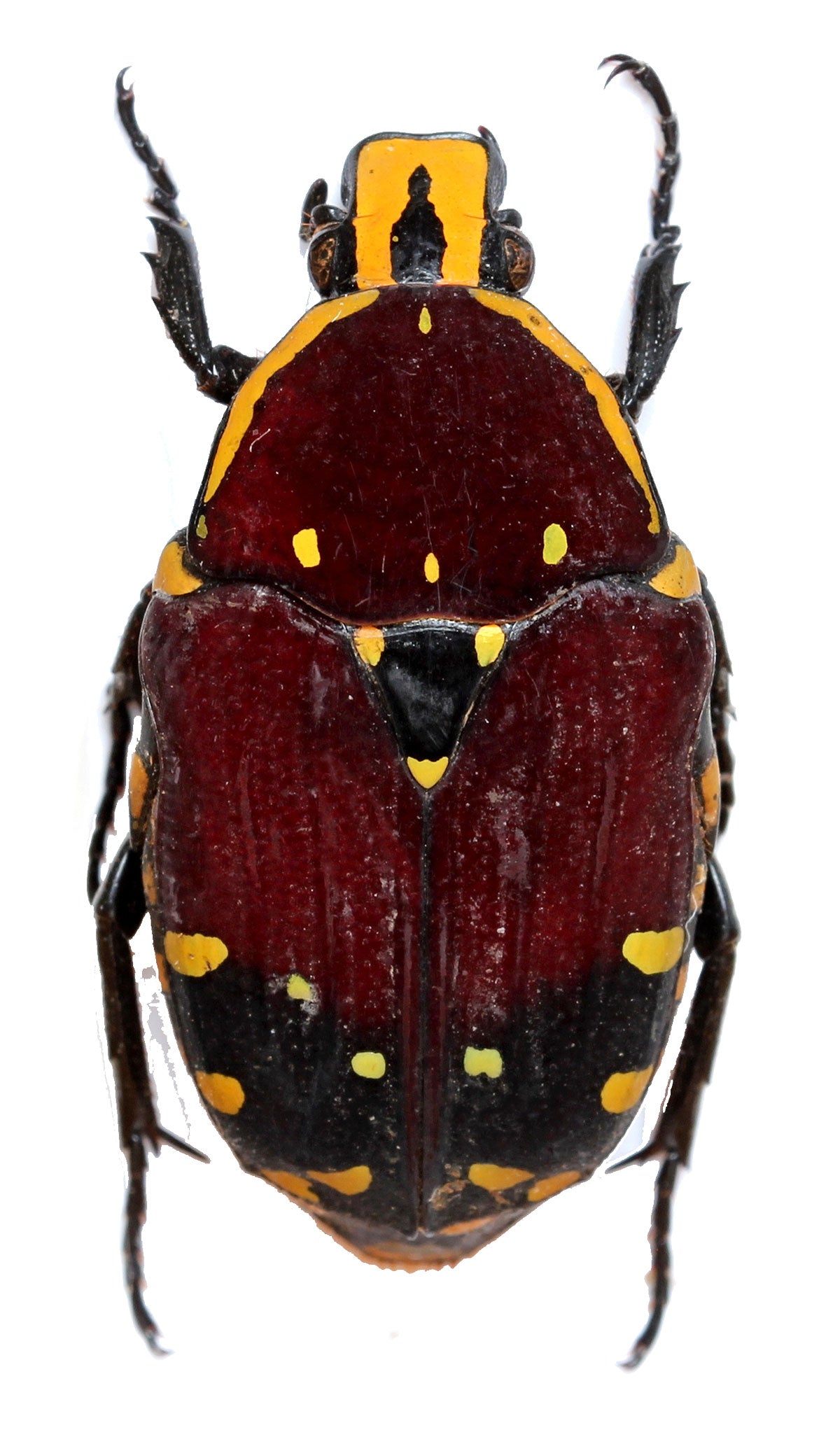The image features a close-up of a beetle against a little white background. The beetle has a distinctive yellow and black squarish head with small eyes on either side. Its head also features small, likely functional chompers, and a notable black marking in the center. The beetle's body is a combination of an oval-shaped brown shell and a yellowish-orange midsection, dotted with distinct yellow spots arranged in segmented sections. Its back is predominantly red with some black regions towards the bottom, and it lacks wings, indicating a hard outer shell instead. Six black legs, which appear pointy and slightly hairy, extend from its body, enhancing its intricate appearance. Despite the ambiguity of the scale and visual detail, the close-up provides a vivid, detailed view of this large beetle.